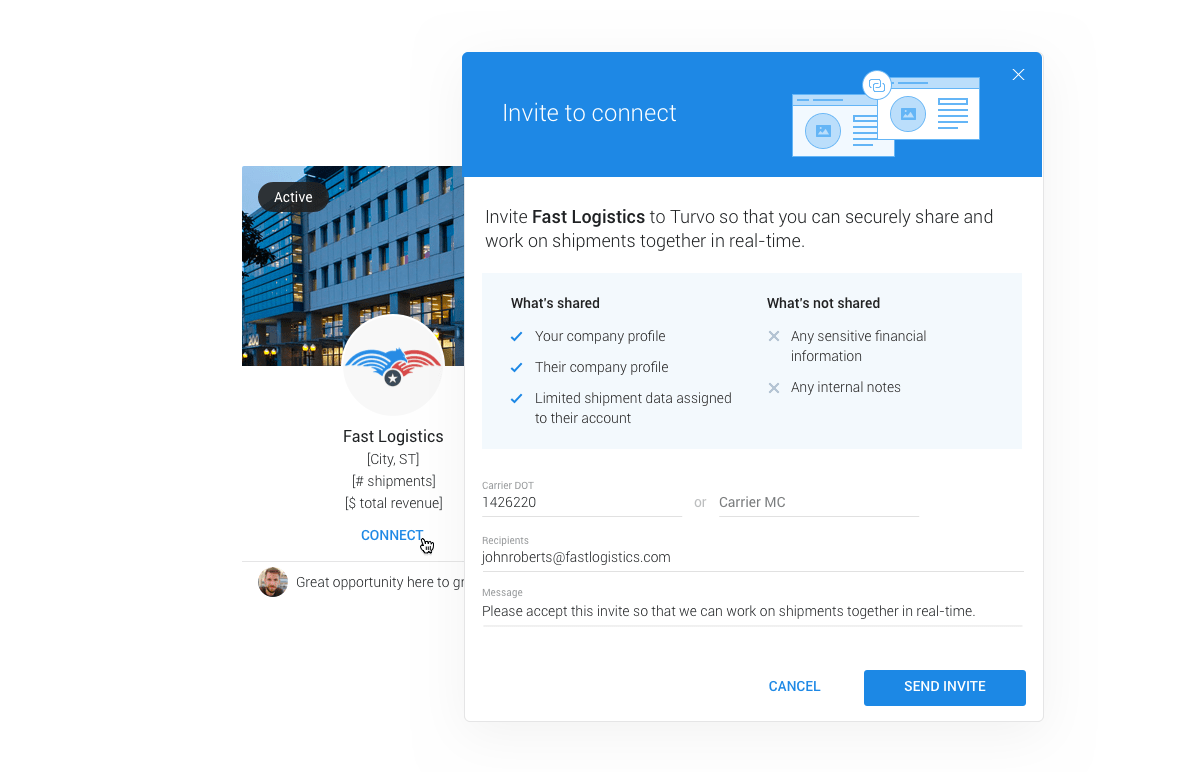This screenshot features two distinct images side by side. The larger, square-shaped image on the right is framed by a blue banner at the top, which contains white text that reads "Invite to Connect." This banner is adorned with generic clip-art style cartoons in blue and white hues, depicting boxes with circles and lines. Below the banner, the rest of the image background is white, with black text stating, "Invite Fast Logistics to Turbo so that you can securely share and work on shipments together in real time." Further down, the image includes a section detailing 'What's Shared' and 'What's Not Shared.' Items under 'What's Shared' are marked with a green check mark and include the company's profile, while items under 'What's Not Shared,' marked with an X, include internet notes, emails, and messages.

The smaller image on the left, positioned adjacent to the larger one, follows a blue and white color theme. It prominently features the logo for Fast Logistics, which is designed within a white circle. The logo showcases a stylized blue and red bird-like cartoon character, which presents a playful and dynamic visual identity, accompanied by a smaller white star encapsulated within a circle.